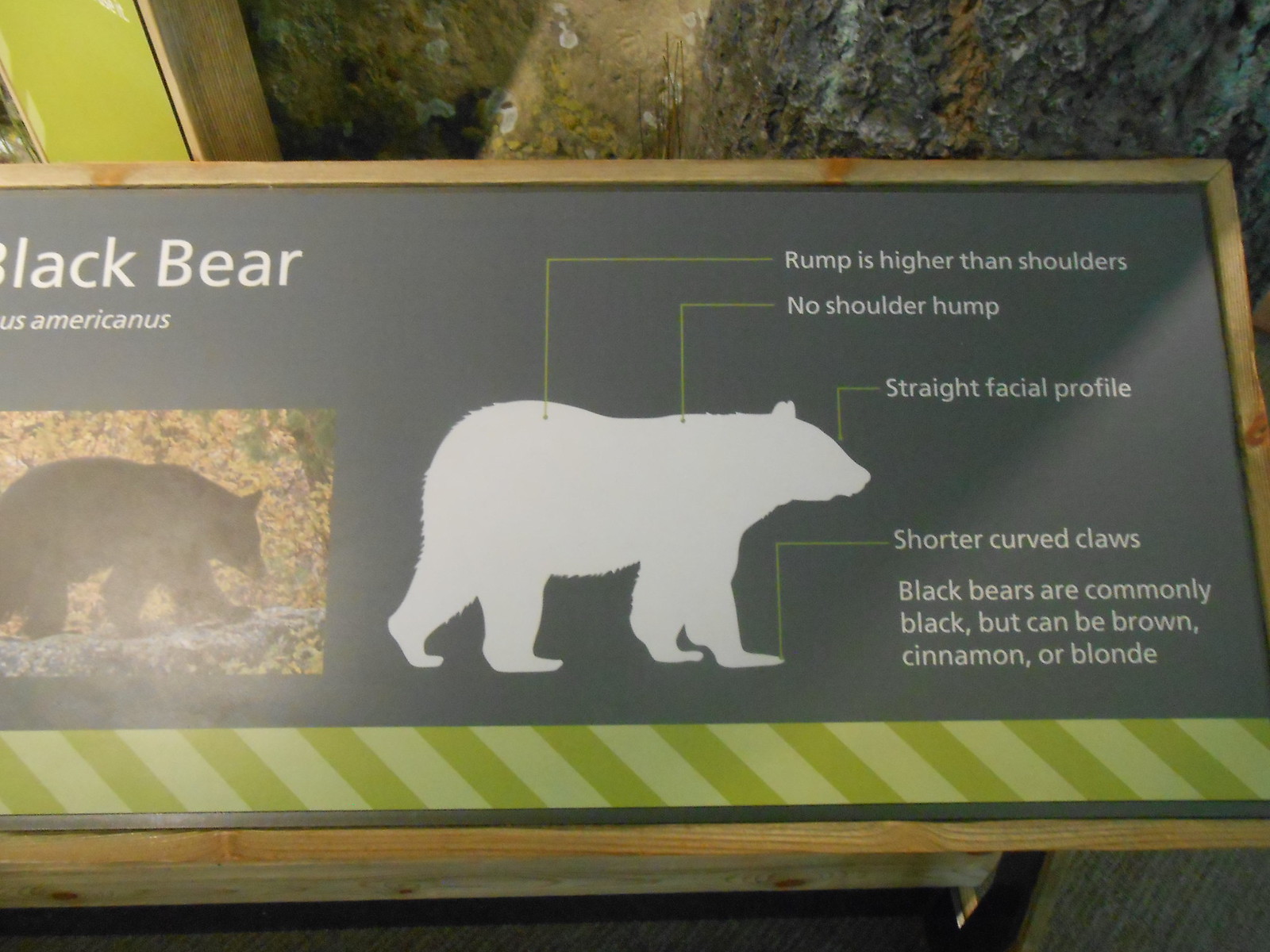The image depicts an educational sign about black bears, centrally positioned within a wooden frame. In the background, there are glimpses of trees and glass, suggesting the setting is outdoors, potentially at a zoo, near a black bear exhibit. The sign features a photograph of a black bear walking on all fours in the left corner and a white silhouette sketch of the bear on the right. Green lines extend from the bear sketch with white captions indicating key characteristics: "rump is higher than shoulders," "no shoulder hump," "straight facial profile," and "shorter curved claws." The sign notes that while black bears are commonly black, their fur can also be brown, cinnamon, or blonde. The overall color scheme includes shades of green, gray, black, brown, and white.